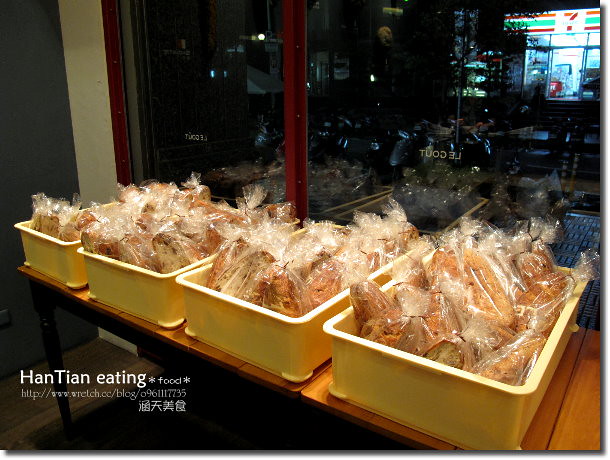The photograph, taken at night inside a building, showcases a well-lit, bustling scene. The focal point is a light brown wooden table supported by black legs, staged in front of a large glass window. On the table sit four yellow bins filled with bagged food items, specifically small loaves of bread and sub-sandwiches wrapped in clear plastic. The window reveals a night view of a brightly illuminated 7-Eleven sign across the street, with its iconic red, orange, and green horizontal lines clearly visible. Additional context includes a small fleet of motorcycles parked outside, adding a layer of urban vibrancy to the scene. On the bottom left of the image, the logo of Han Tian Eating, along with a website and some Chinese characters, is prominently displayed, reversed due to the perspective. The window itself has a reddish border, further framing the scene inside and out.